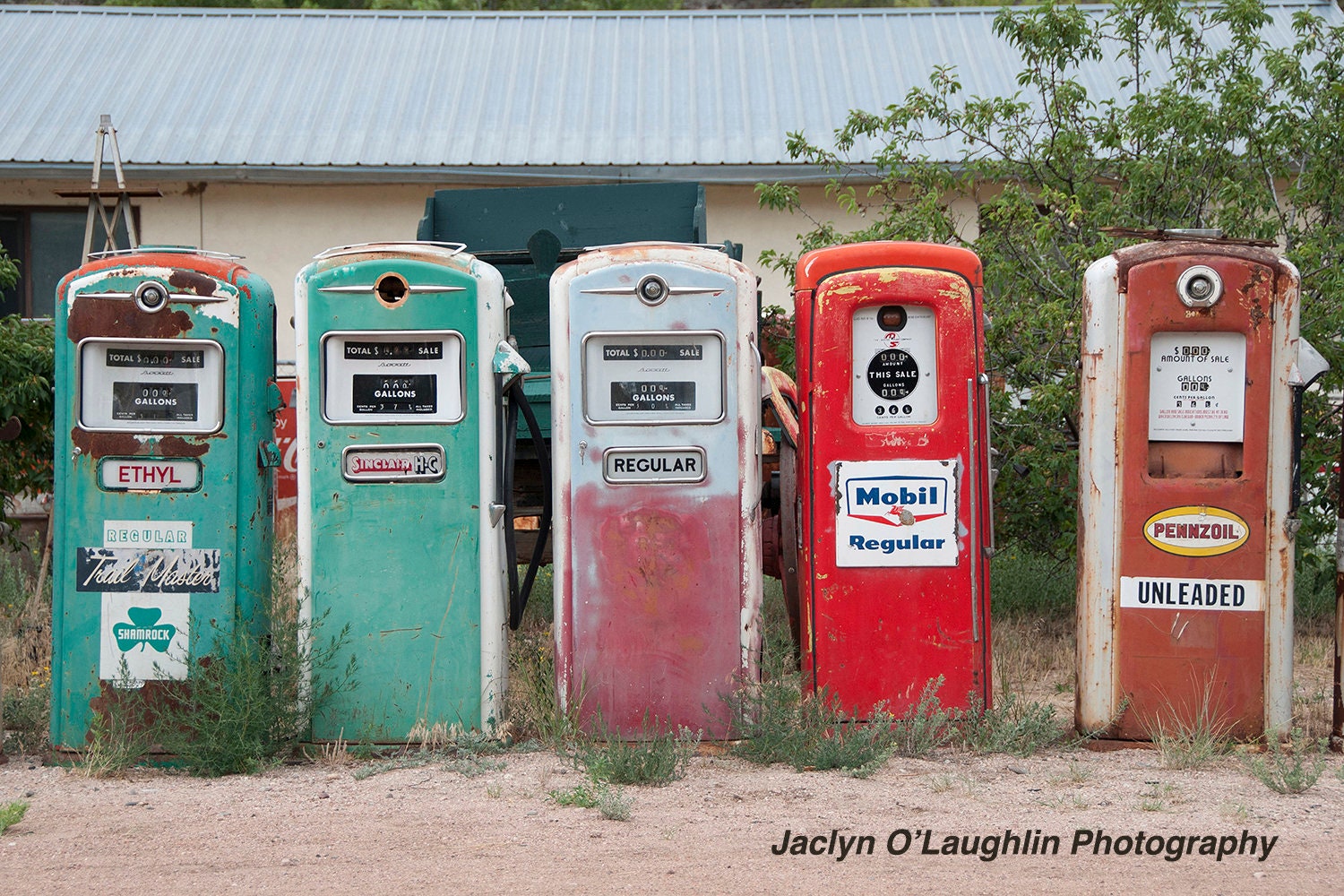This color photograph by Jacqueline O'Loughlin captures a striking lineup of five antique gas pumps set outdoors on a sandy, weedy ground. From left to right, the first green pump proudly brandishes the Shamrock logo with "Ethel" and "Regular" in red text. Next to it stands a green Sinclair pump. At the center is a faded red and white pump with "Regular" written in black text. The fourth pump is a vibrant red with the word "Mobil" and "Regular" displayed in blue and red text. The fifth and final pump is a distinctive brick-orange Pennzoil pump, marked "Unleaded" in a mix of white, yellow, and red text. Behind these vintage relics lies a long building with a blue slanted roof, accompanied by an old green wooden wagon and partially shaded by a nearby bush and tree.